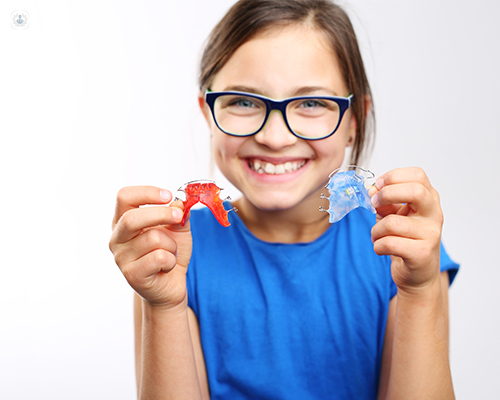The image is a rectangular photograph with a young girl positioned at its center against a white backdrop. She is smiling brightly, showcasing her teeth while wearing large, black-rimmed glasses. Her brown hair is neatly pulled back into a ponytail. Dressed in a short-sleeved blue shirt, the girl is visible from her stomach upwards. She holds up two teeth retainers: a red one in her right hand and a blue one in her left. A grey wreath encircling a small green outline of a person's head and upper shoulders serves as a watermark in the top left corner, hinting at a dentistry setting. The overall mood is one of excitement and pride, likely related to her dental care journey.